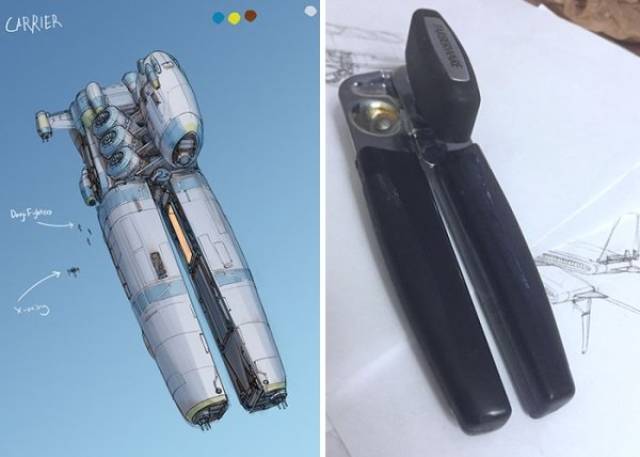The image features a dual composition of identically sized vertical rectangles. On the left side, there is an engineering rendering of a can opener against a gradient blue background. The top left of the rendering has the handwritten label "CARRIER" in white, all-caps lettering. In the top right corner of this image are four horizontal dots: blue, yellow, red, and light gray. The drawing depicts the can opener in a top view, highlighting its silver or gray metallic structure with buttons and gears, and some blue stripes on its separated halves. White handwritten notes with arrows are pointing towards different parts of the can opener.

The right-side image shows a photograph of a real can opener that closely resembles the mechanical drawing. This can opener is placed on a white surface, angled similarly to the rendered version from top left to bottom right. It has a black handle and silver metal components, including the gear mechanism and a silver plate on the hand crank, which features a small, unreadable logo or brand name in black. The can opener in the photograph is positioned on an open book with blank pages and scribbles. This meticulous comparison shows the real can opener mirroring the detailed futuristic and mechanical aspects of the rendering on the left.